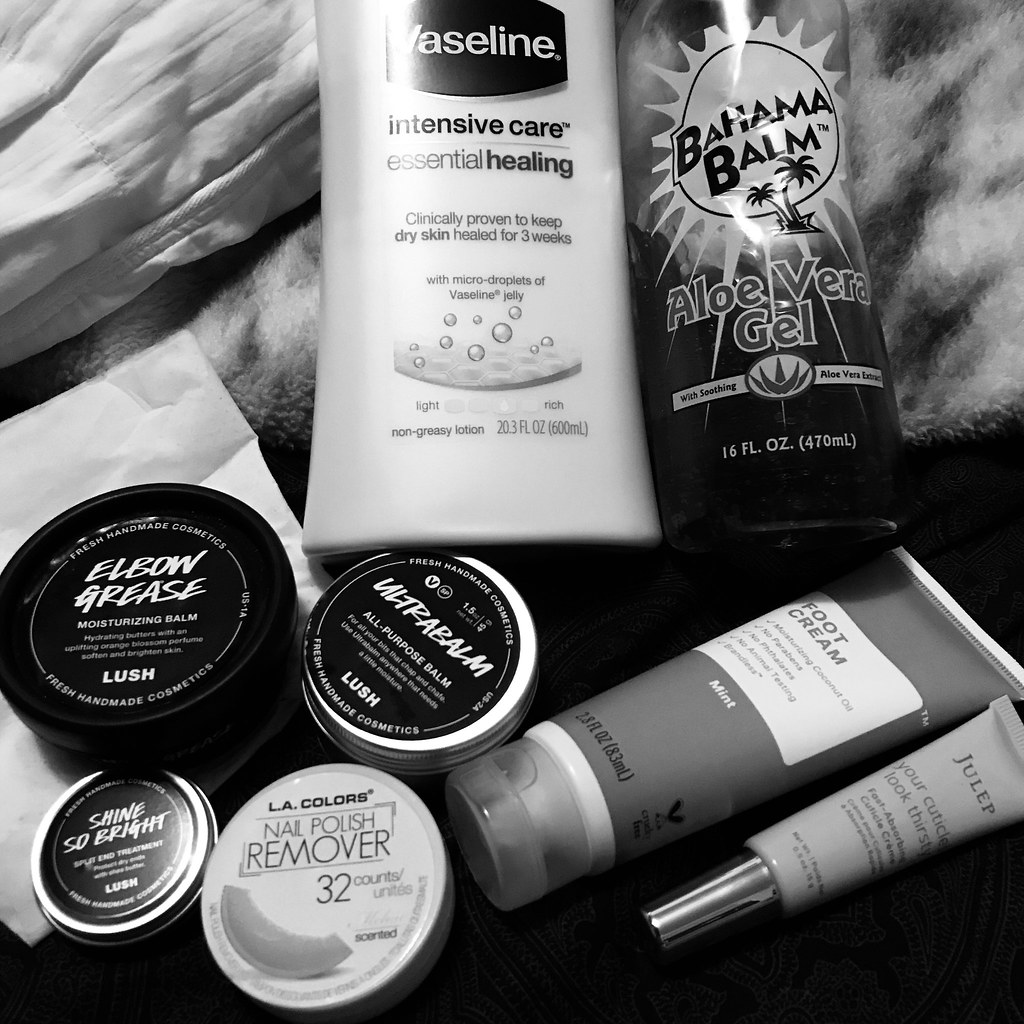A meticulously arranged black and white photograph captures an assortment of beauty products on various fabric textures. The top left corner displays the edge of a comforter extending diagonally about two inches into the space, overlaying a fluffy, white and black quilt that occupies the upper middle section. Below, the lower half of the image reveals a slick, black sheet, creating a dramatic backdrop.

Emerging from the left and positioned over both the comforter and quilt, a half bottle of Vaseline Intensive Care lotion commands attention. This bottle, extending slightly past the midway point vertically, is predominantly white with a large black square in the center, which contains the brand name "Vaseline" in white letters, accompanied by additional product details below.

To the right of the Vaseline bottle, a partially full transparent bottle peaks from the top edge of the frame, its bottom aligned with the Vaseline’s midpoint. The bottle features a sun icon with rays, labeled "Bahama Balm Aloe Vera Gel."

Descending to the left side, past the halfway mark, a round, black tub reminiscent of a hockey puck stands out with "Elbon Elbow Grease” marked in white letters, surrounded by further descriptive text. This tub rests on a white piece of paper angled up from the left and extending to the right before sharply descending off the bottom edge, creating a contrasting platform.

Beneath the elbow grease jar, a small, flat container with a silver border and black center displays the word "Shine" in white text. To the direct right of this container lies a slightly larger, similar styled case marked "Ultra Balm."

Further below, a small, white container reveals a banana graphic in the bottom left corner and is labeled "LA Colors," with additional lettering adorning the surface. To the upper right of this container, a squeezy bottle with a clear cap leans at an angle, marked "Foot Cream" in a white square. Below it, another smaller squeezy bottle mirrors the same tilt, showcasing a silver cap and white body embellished with black lettering.

This carefully curated collection of beauty essentials, juxtaposed on various textured fabrics, creates a visually appealing and detailed tableau.